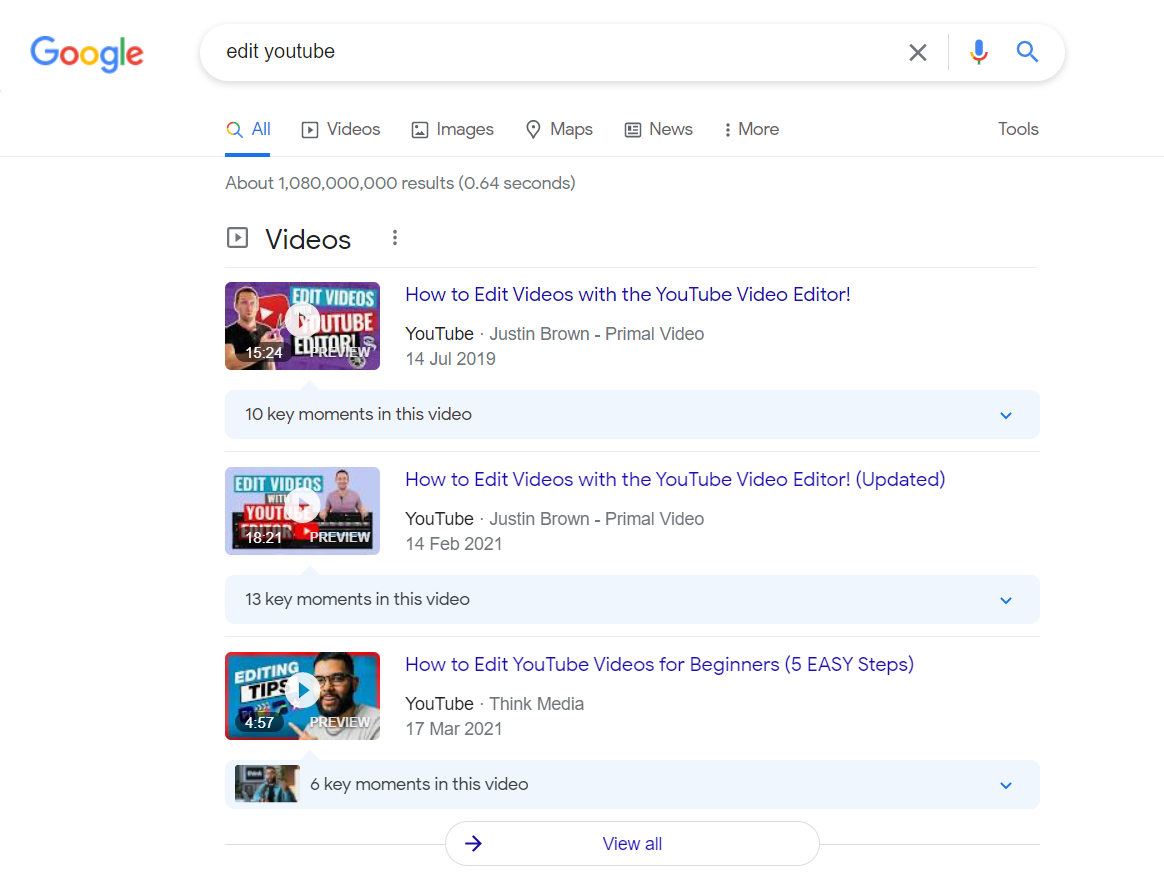The image depicts a Google search results page on a computer. The query "edit YouTube" has been entered into the search bar. Beneath the search bar, a navigation menu features options for "All," "Videos," "Images," "Maps," "News," and "More." The search has returned approximately 1,080,000,000 results, displayed within 0.64 seconds. 

Scrolling down, the first listed video result is titled "How to Edit Videos with the YouTube Video Editor," which highlights "10 key moments in this video." Further down, another video titled "How to Edit Videos with Your YouTube Video Editor - Updated" appears, showcasing "13 key moments in this video." Continuing down the page, a video titled "How to Edit YouTube Videos for Beginners: 5 Easy Steps" is displayed, featuring "6 key moments in this video."

At the bottom of the video listings, there's a "View All" button. Additionally, the search bar is equipped with icons for voice search (a microphone), search suggestions (an X to clear the search), and the traditional magnifying glass for initiating searches.